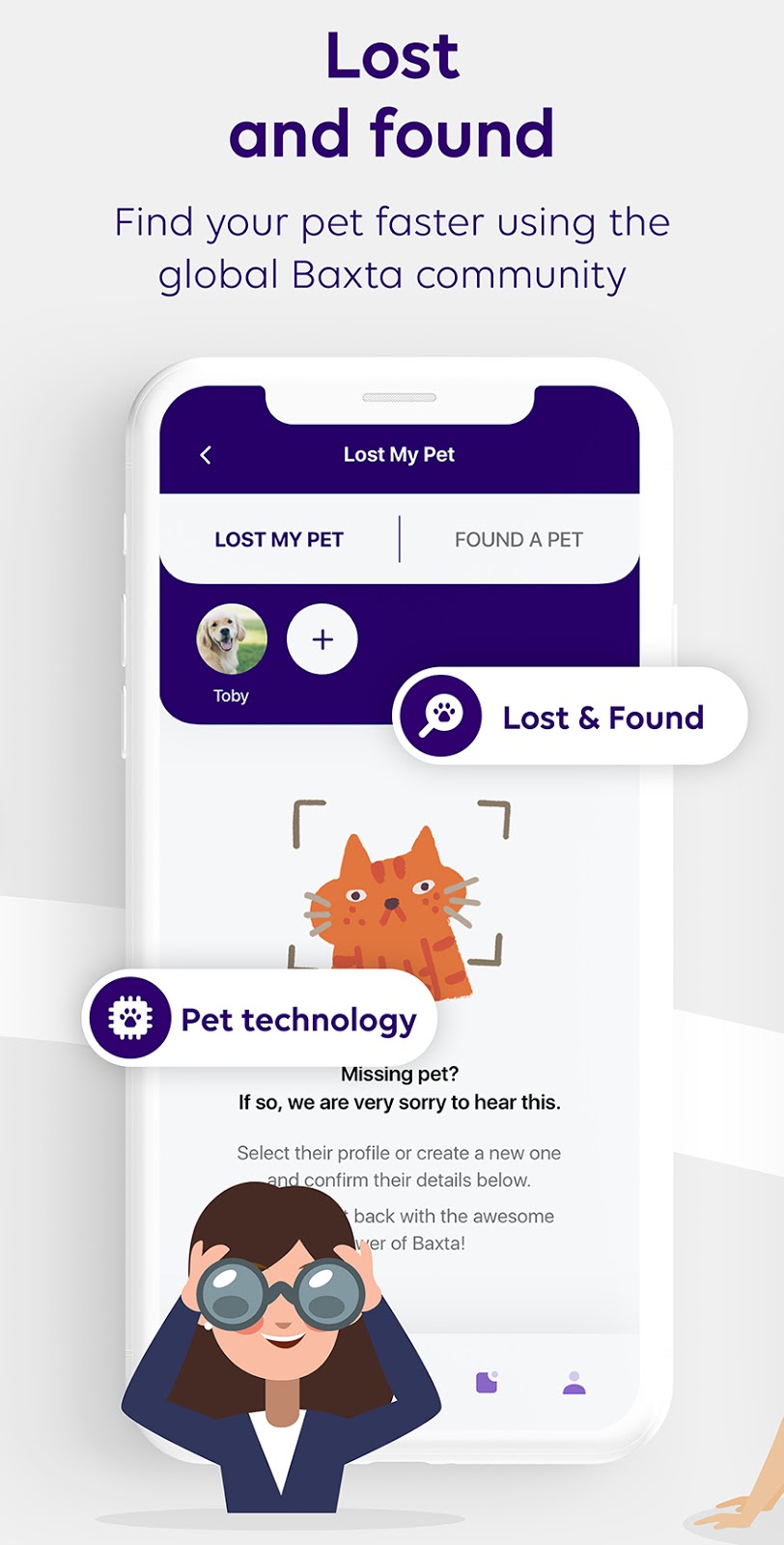The image is a color, computer-generated advertisement designed to promote a mobile app called "Lost My Pet." The advertisement primarily features a detailed depiction of the app displayed on a smartphone. The phone screen shows the "Lost My Pet" tab active, highlighting a specific lost pet profile. The profile belongs to a dog named Toby, who appears to be a golden retriever. The screen also features text that reads: "Missing Pet. If so, we are very sorry to hear this. Select their profile or create a new one to confirm their details below." This message emphasizes the app's function of helping users publicize their lost pets and update the community once the pet is found.

Above the smartphone, blue text reads: "Lost and Found. Find your pet faster using the global Baxter community." The name "Baxter" is presumed to be the name of the app or the community it supports. Other text elements include "pet technology," reinforcing the advanced technological aspect of the service. Additionally, there is an overlay icon and further "Lost and Found" text incorporated into the design.

In the bottom left corner of the advertisement, there's an illustration of a woman, portrayed in a cartoon style, looking directly at the viewer with goggles on, symbolizing the active search for lost pets. This element adds a human touch and an engaging visual cue to the advertisement, making it more relatable and visually appealing.